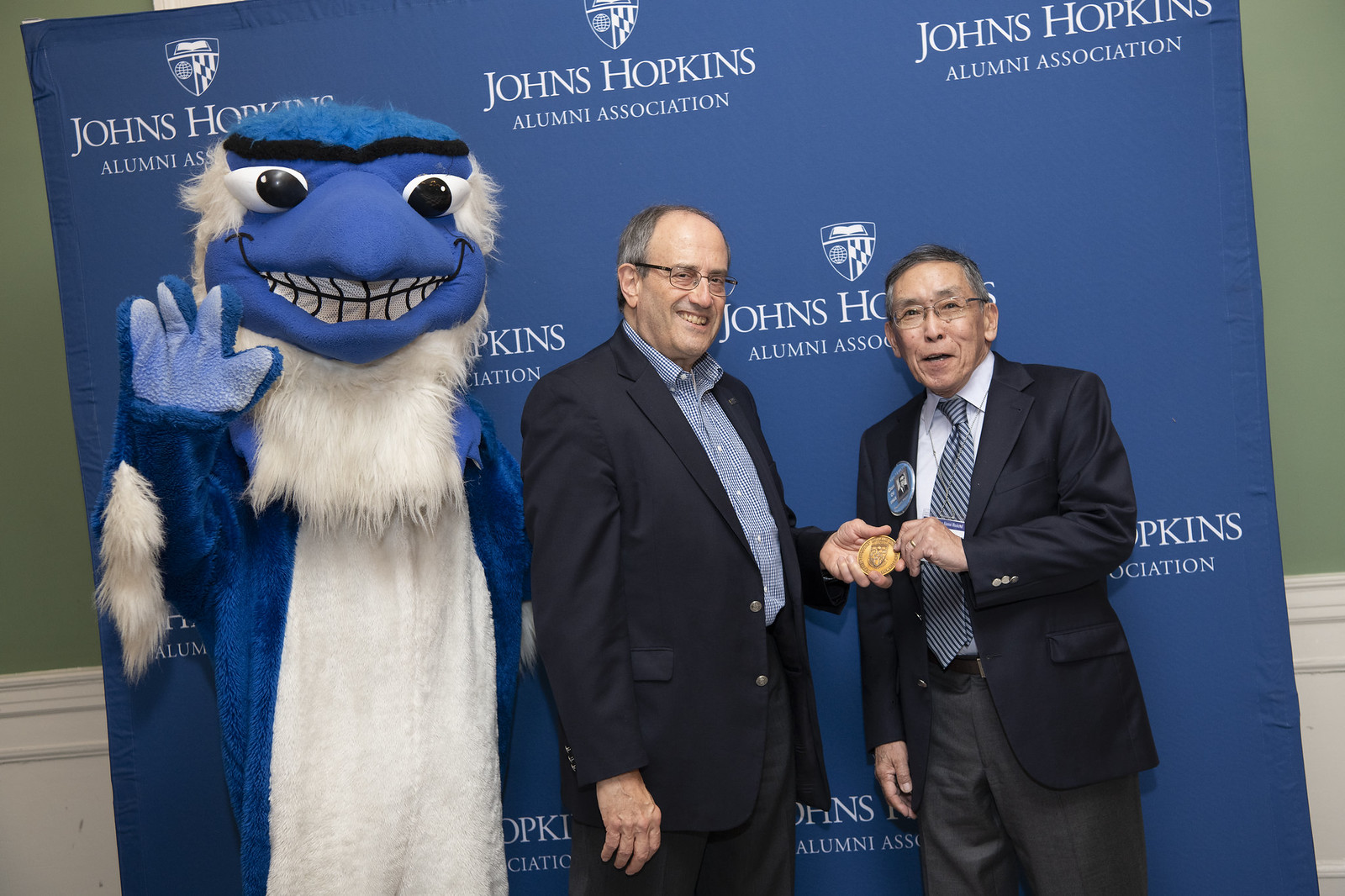The image depicts an indoor setting featuring three individuals prominently positioned at the center. On the far left is a tall mascot resembling a bird, identifiable by its blue and white costume and distinctive beak. To its right stand two men dressed in formal attire. The man in the middle, who is balding and wears a suit jacket over a blue shirt with no tie, smiles as he either receives or hands over a circular, somewhat oblong-shaped award. The shorter man on the far right, also in a suit but distinguished by a striped tie, white shirt, and gray pants, reciprocates the action. Both men are wearing eyeglasses. They stand in front of a blue backdrop adorned with the "John Hopkins Alumni Association" text and accompanying shield logo. The color palette of the scene includes green, white, blue, black, and gray, and the setup suggests the photograph was taken during an award ceremony or a formal gathering.